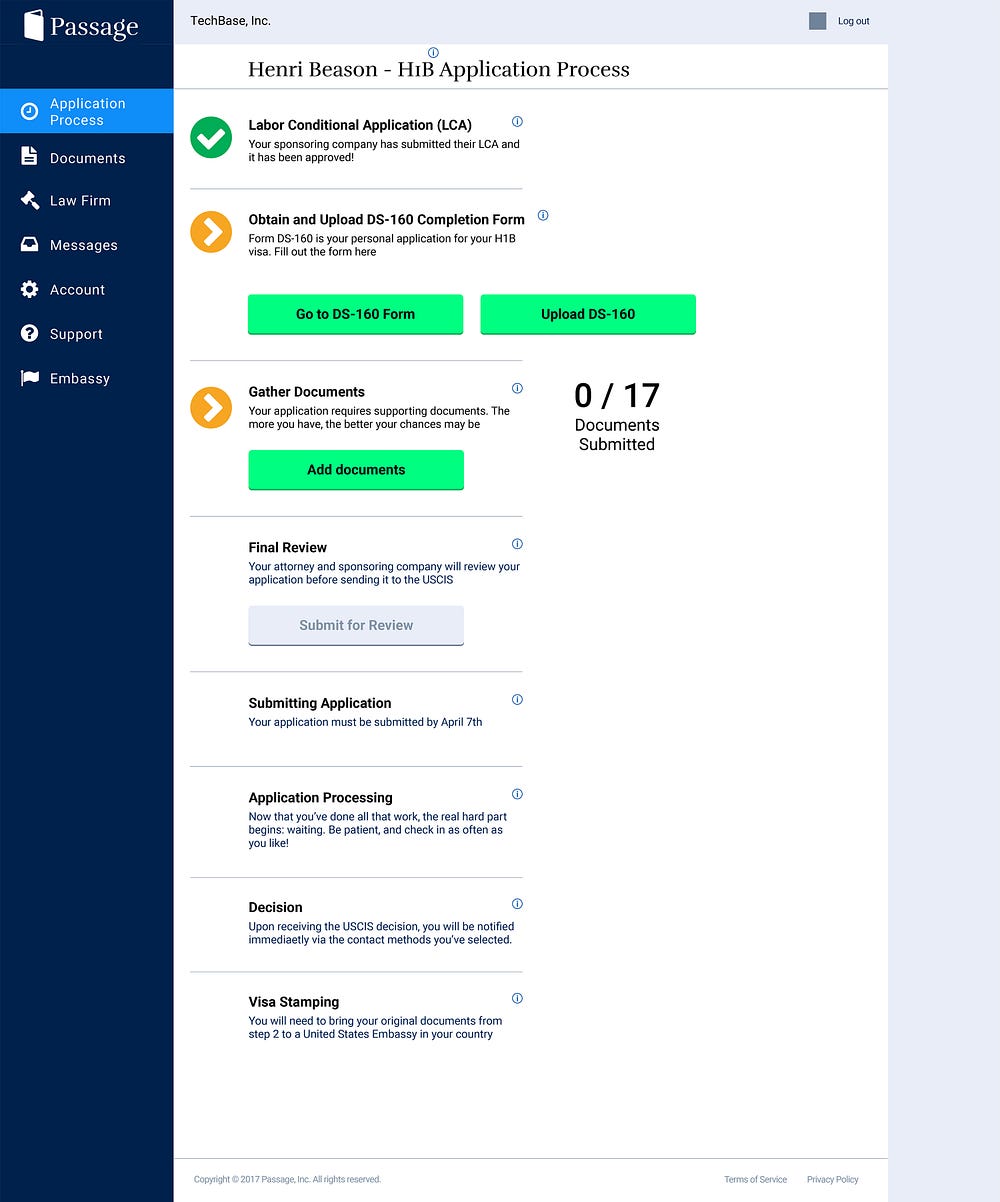**Detailed Caption:**

This image is a vertical screenshot of a website interface. At the upper left-hand corner, it displays the website name "Passage" accompanied by a white book icon on its left. The layout is split into three parts: a vertical dark blue border on the left with various headings, a central section with a white background, and a gray vertical border on the right-hand side.

At the top of the website, there is a light gray banner bar that reads "Techbase Inc." with a logout icon located at the upper right-hand corner. The left vertical dark blue border features a highlighted heading titled "Application Process". Below this, the headings listed include "Application Process," "Documents," "Law Firm," "Messages," "About," "Support," and "Embassy."

The main central section of the screen is dedicated to the title "Henry Beeson's HIV Application Process." This section contains step-by-step instructions moving from top to bottom, divided into distinct categories:
1. Labor Conditional Application (LCA) - Indicated complete with a green check mark.
2. Obtain and Upload DS-160 Completion Form - Accompanied by a yellow button with a right-pointing arrow.
3. Gather Documents - Similarly marked with a yellow button with a right-pointing arrow.
4. Final Review
5. Submitting Application
6. Application Processing
7. Decision and Visa Stamping

The interface indicates that 0 out of 17 documents have been submitted. In the section for "Obtain and Upload DS-160 Completion Form," light green buttons are available labeled "Go to DS-160 Form" and "Upload DS-160." Under the "Gather Documents" heading, there is a green button labeled "Add Documents."

This detailed caption attempts to provide a clear visual and functional understanding of the website's interface as depicted in the screenshot.